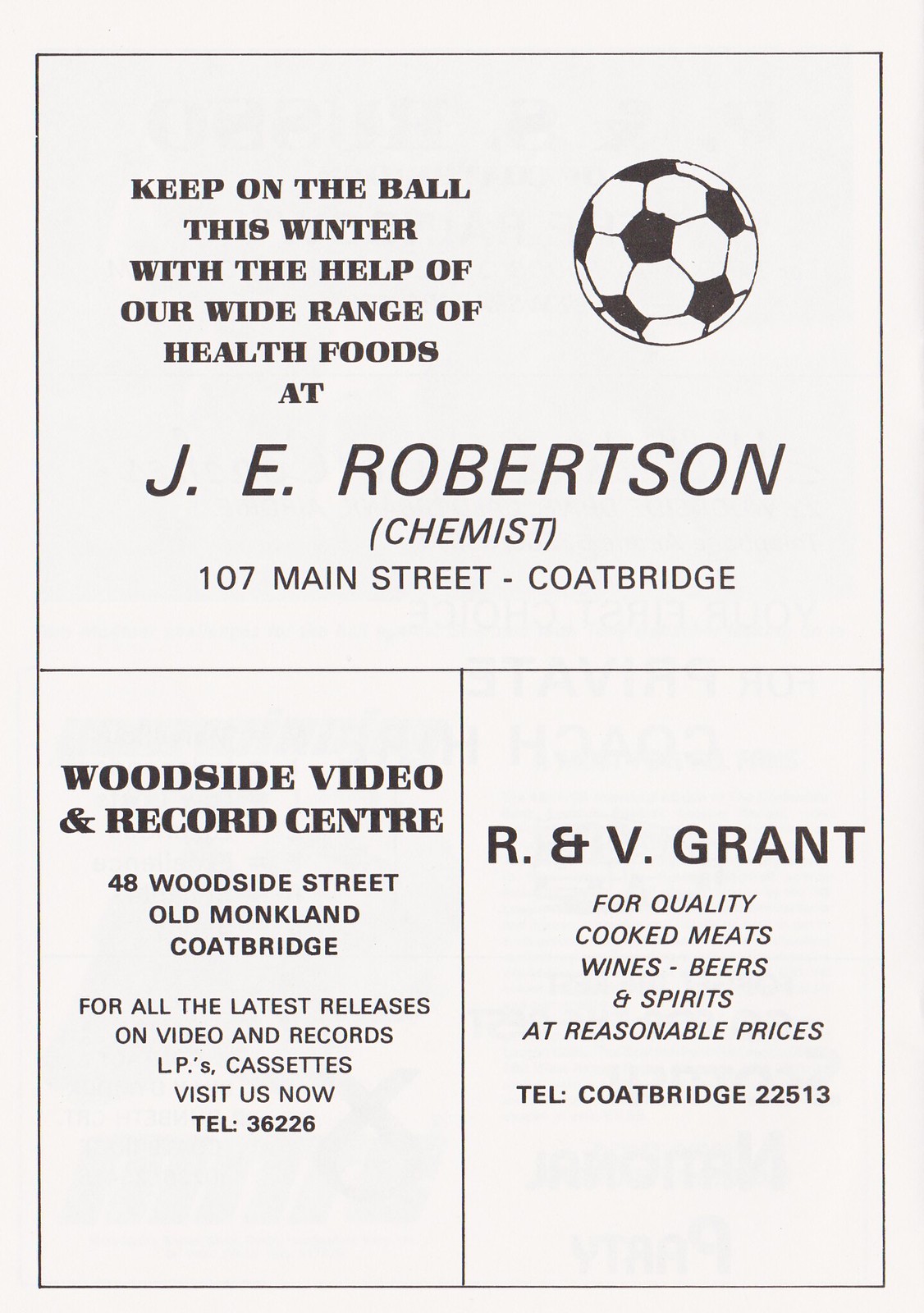This image depicts a promotional poster divided into three sections against a light grey background, with black text in each section. The top section, taking up roughly half of the poster, features the slogan, "Keep on the ball this winter with the help of our wide range of health foods at J.E. Robertson Chemist, 107 Main Street, Coatbridge." This section also includes an illustration of a black and white soccer ball to the right of the text. 

The bottom half of the poster is split into two equal rectangular sections. The left section advertises the "Woodside Video and Record Center, 48 Woodside Street, Old Monk Land, Coatbridge," offering "all the latest releases on video, records, LPs, and cassettes," with the contact number "Tel 36226." 

The right section promotes "R&V Grant" known for "quality cooked meats, wines, beers, and spirits at reasonable prices," with the contact number "Tel Coatbridge 22513."